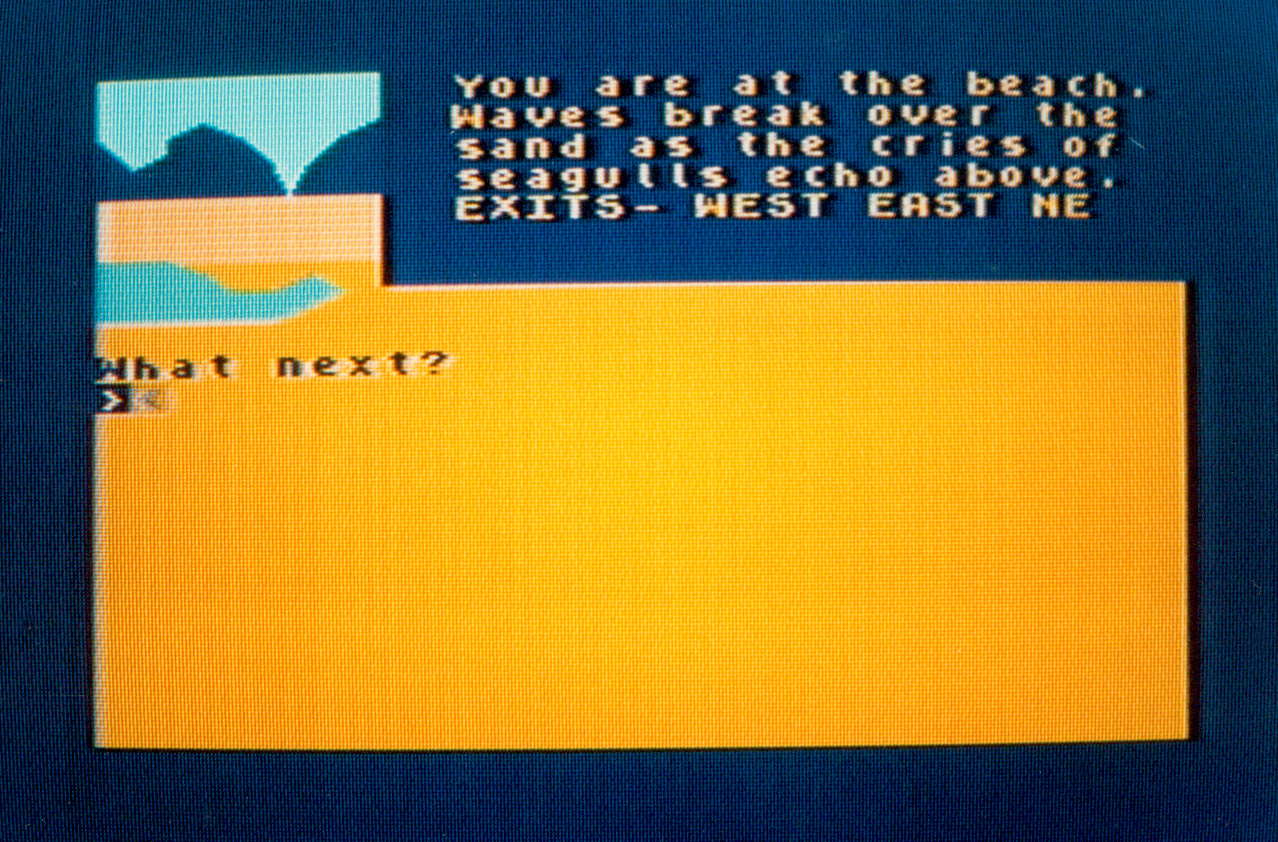We are looking at a letterboxed screenshot from a vintage, mid-to-late 80s-style text adventure video game. The image's overall dimensions are roughly 30% wider than it is tall, framed by a royal blue border that occupies about 5-10% of the outer edges. The main display area contains a large yellow box centrally located on the screen, which appears pixelated in design. Within this yellow box, at the top left, there is a graphical rendering—likely a low-resolution depiction—showing some blue water and mountains in the background. 

The top portion of the yellow box houses a block of text in orange letters that reads, "You are at the beach; waves break over the sand as the cries of seagulls echo above." Beneath this description, a line of text in all caps states, "EXITS: west, east, northeast." Below this, the prompt "What next?" invites user interaction, indicating a space for typing commands in the center-left area of the yellow box. The entire interface exudes a nostalgic feel, reminiscent of early computer adventure games, combining minimalistic pixel art with text-based navigation cues.